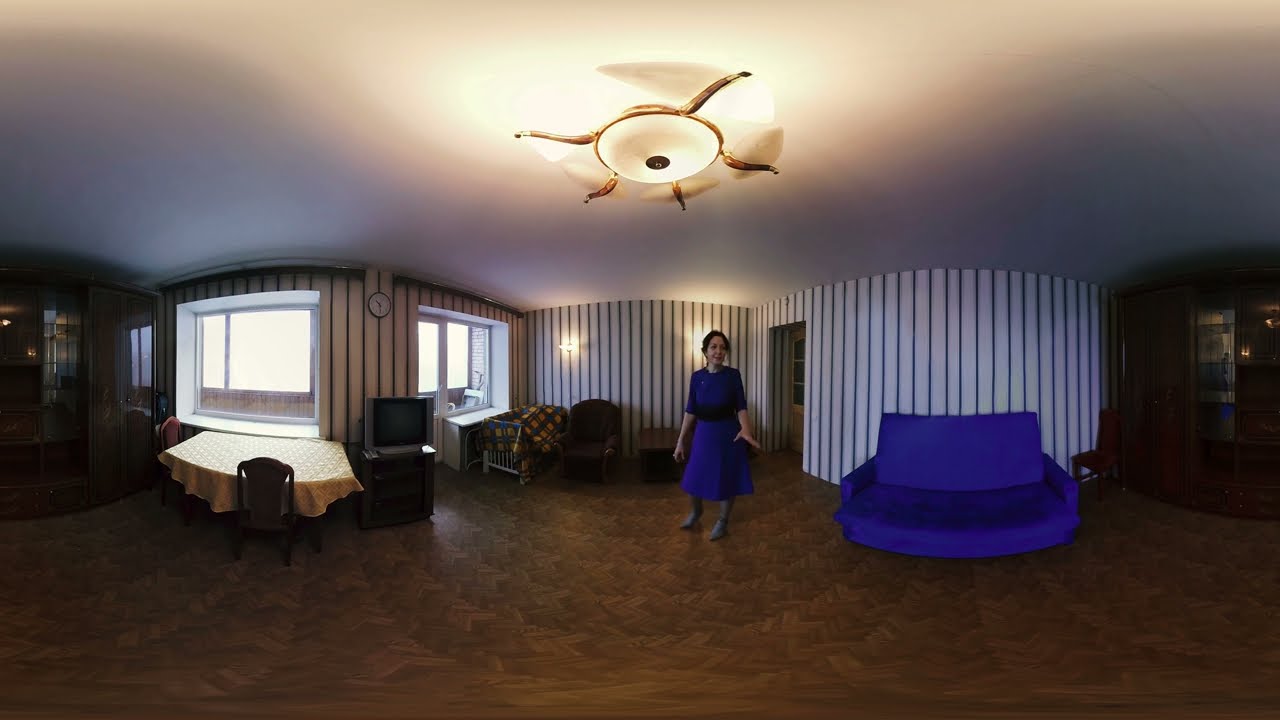The image depicts an elaborately designed room with a warped, almost panoramic quality that makes it appear as if viewed through a peephole. At the center, there's a woman in a knee-length blue dress, featuring quarter-length sleeves and a black belt. She has dark hair and is wearing gray leggings or tights paired with gray boots. The woman is gesturing with her hands, looking off to the side.

On the right side of the image, there's a blue, slightly curved sofa. Adjacent to it is a small red chair with wooden sides and a matching hutch, made of wood with see-through windows. The flooring throughout the room is a designer tile in a wooden color.

The walls are distinct, featuring varying designs: some are white with black stripes, and others are beige with black stripes. Two large glass windows flank the room, allowing natural light to filter in. Positioned beside one of the windows is a baby crib with a plaid blanket in blue, yellow, and red colors, located next to a peculiar, brown single sofa chair.

On the left side of the image, a flat-screen TV rests atop a brown TV stand near a window. Above the TV, a circular clock displays 10:30. There is also a large brown hutch with windows and a brown-table-dining setup, which includes a table covered with a yellow tablecloth and surrounded by reddish-brown chairs. Additional furniture includes a brown table and another hutch on the right side of the sofa.

The ceiling is white, adorned with a designer light featuring a gold design around its translucent center. The room exudes a clash of styles, adding to its intriguing and complex visual appeal.